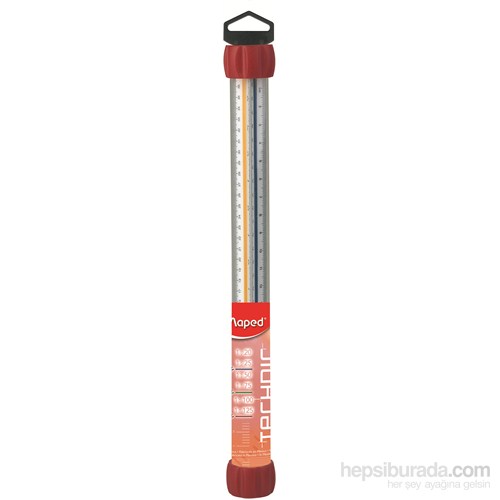The image displays a thermometer-like measuring instrument with distinct, colorful features. The main component is a cylindrical measuring stick adorned with numerical markings along its side, indicating its measuring capability. At the top of the tube is a black handle with a white cutout section. Beneath this handle, a prominent red lid separates the upper black segment from the measuring stick. The measuring stick itself features two vertical stripes—one yellow and one blue—extending down its length.

Below these vibrant stripes, the tube's color transitions into a light peachy pink shade. Along this section, there is vertical text; however, the letters are partially obscured, making them difficult to read. The base of the thermometer-like device is capped with a dark brown plug, completing its structure. The variety of colors and elements make the instrument visually distinctive and complex.